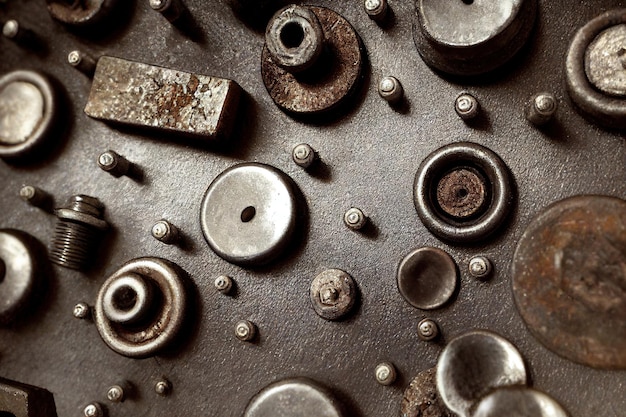The image is a detailed close-up of a rough, dark metal surface, possibly a workbench or an artistic representation resembling a steampunk aesthetic. Scattered across the surface are various mechanical components, predominantly circular or cylindrical in shape, including nuts, bolts, washers, rivets, and screws of different sizes and conditions. Dominating the left side, an overturned nut reveals its threading. There are approximately 30 to 40 metal items visible, many of which exhibit signs of wear, with rust being a prominent feature. A rectangular, ramp-like piece with a rusted appearance is situated near the center, while a larger, cylindrical, and stacked component lies toward the lower half. Several polished and corroded metal disks and knobs create a contrast against the dark, patinaed background. The overall arrangement of the objects seems random, contributing to the chaotic yet intriguing visual composition.